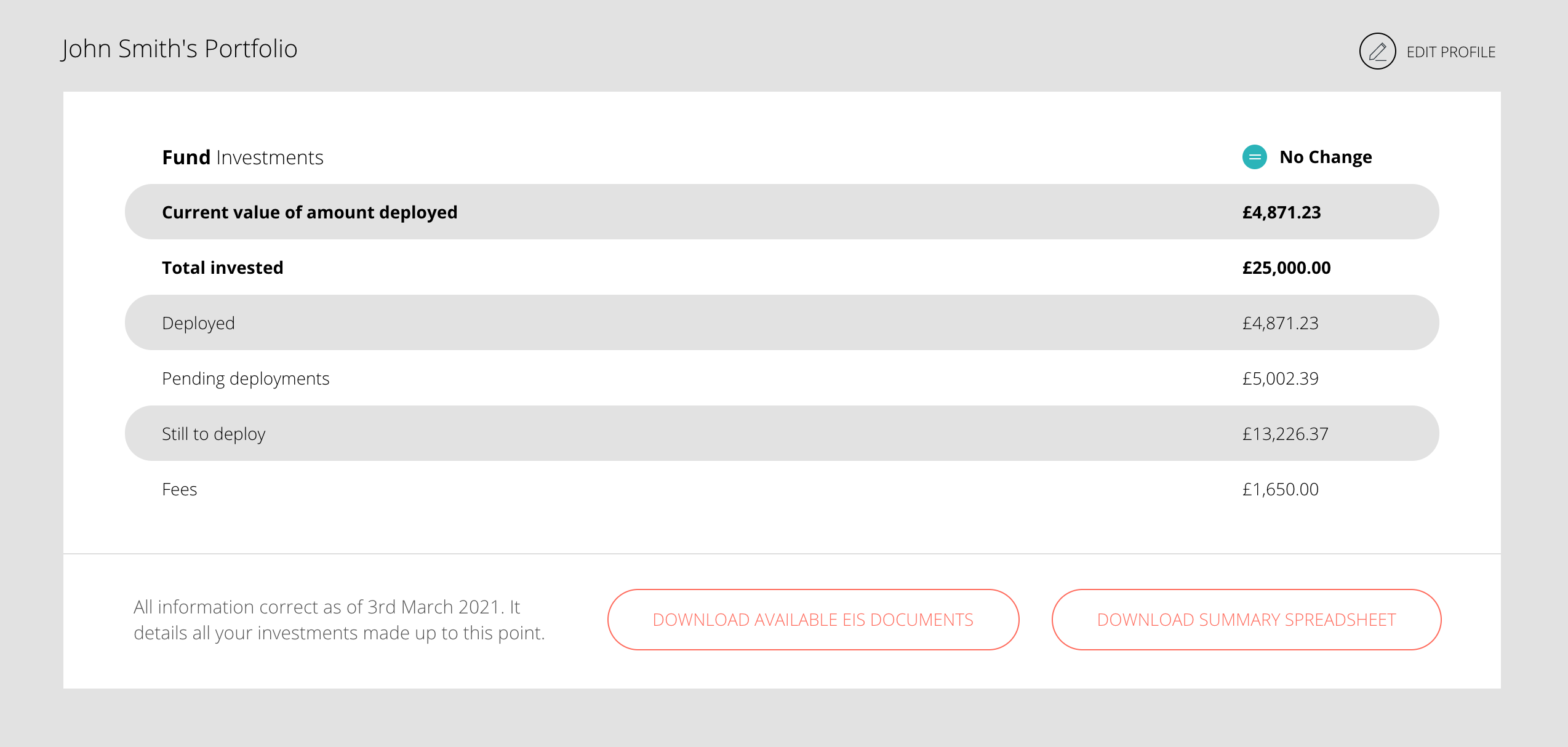This horizontally oriented rectangular screenshot is enclosed by a gray border. In the top left corner, in black text, it reads “John Smith's Portfolio.” On the top right, there is a circular icon featuring a pencil in the center, next to the text “Edit Profile.” The central background of the image is white, featuring detailed textual information about John Smith's fund investments. 

The key figures highlighted include:
- "Fund investments: No change" 
- "Current value of amount deployed: £4,871.23"
- "Total invested: £25,000"
- "Deployed: £4,871.23"
- "Pending deployments: £5,002.39"
- "Still to deploy: £13,226.37"
- "Fees: £1,650"

It concludes with the statement, "All information correct as of 3rd March 2021," detailing all investments made up to this date. 

At the bottom right of the screenshot, there are two wide, oval-shaped buttons outlined in red. They respectively read “Download Available EIS Documents” and “Download Summary Spreadsheets.”